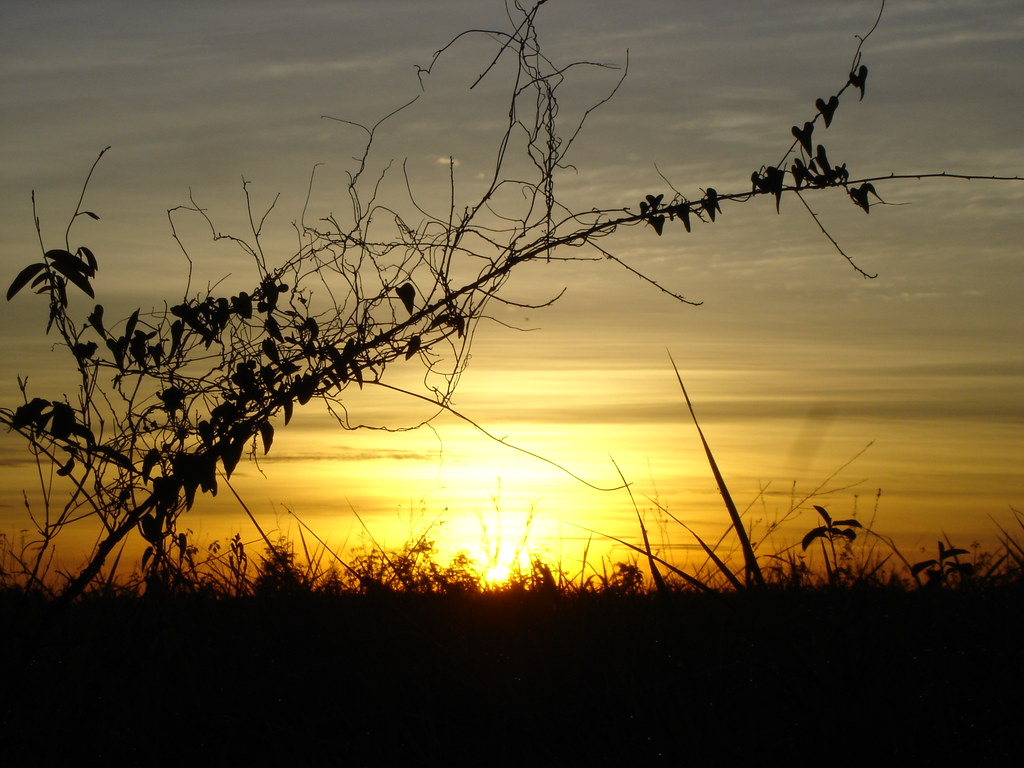In this evocative outdoor scene photographed at sunset, the sun is almost completely set, casting an enchanting glow of yellow and orange across the sky and reflecting brilliantly on the ocean. Shadows fall over a grassy field in the foreground, with tall weeds and sticks protruding upward, creating a silhouetted effect against the vivid evening sky. The field extends from left to right, bathed in the ethereal light of the setting sun. To the left, a nearly bare tree branch with sparse vines and heart-shaped leaves arcs across the image to the top right, its dark silhouette adding a striking contrast to the warm colors of the sunset. Thin, whispering clouds stretch horizontally across the sky, blending into the darkening gray above. The photograph—whether a striking piece of representational art or realistic color illustration—captures the serene yet vibrant transition of day into night, with every element accentuated by the glowing horizon and reflected on the water's surface.